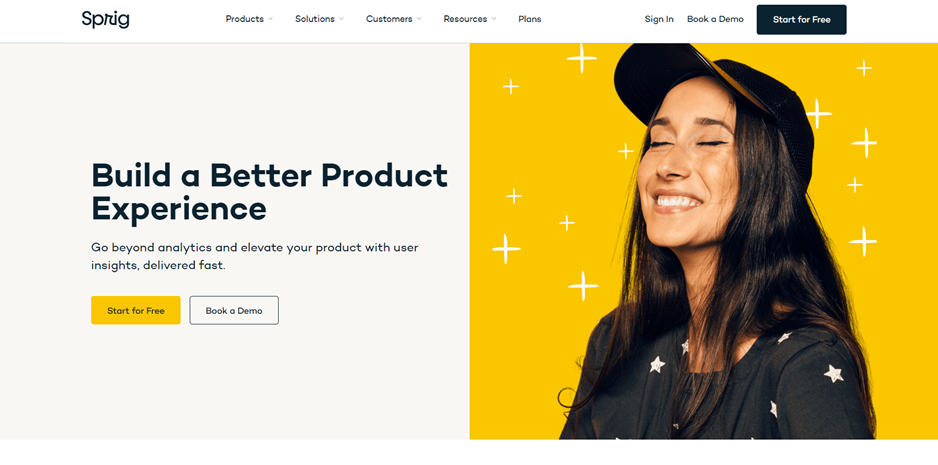Screenshot of the "Sprig" website homepage, showcasing its invitation to "Build a better product experience." The interface features a prominent call-to-action encouraging users to “Start for free” and “Book a demo.” The layout is modern and intuitive, reflecting common contemporary UI designs. Dominating the right side of the screen is a cheerful woman, occupying nearly half the visual space. She has long, brown hair cascading from under a black ball cap and is dressed in a black T-shirt adorned with white stars. Her radiant smile reveals bright white teeth, and her eyes are joyfully closed, all set against a vivid yellow background punctuated by subtle cross patterns. The tagline, “Go beyond analytical and evaluate your product with user insights delivered fast,” suggests that the platform aids businesses in leveraging user feedback to enhance their products. Users are invited to begin their journey free of charge, hinting at a potentially valuable tool for product development.